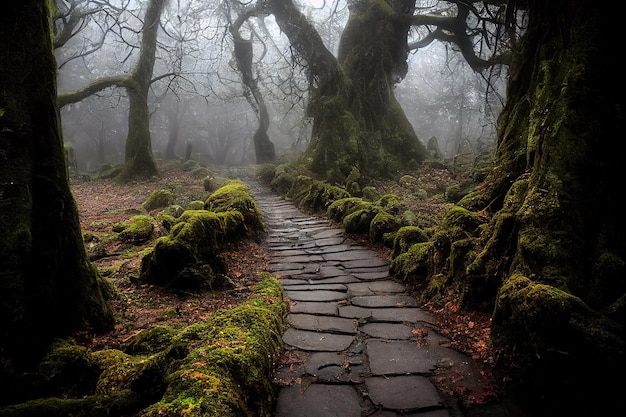In this damp, foggy forest scene, a sense of eerie tranquility pervades the photograph, which is rectangular with its longest edge horizontally aligned. Dominating the left and right sides are large, gnarled trees, their moss-covered branches twisted and intertwined, devoid of leaves. The ground beneath these ancient sentinels is littered with brown, dead leaves and mossy stumps, hinting at a fall setting. Central to the composition is a slightly curved stone path, composed of flat, individually laid stones that meander from the bottom center towards the middle back, gradually veering to the left. Large mossy rocks, some boulder-sized, line the path and add to the dense greenery and overgrowth that characterizes the scene. The atmosphere is heavy with mist and fog, which thickens as it recedes into the distance, creating a moody, almost spooky ambiance. The combination of dark foreground under the canopy of trees and the lighter background shrouded in fog enhances the mysterious allure of this natural landscape.